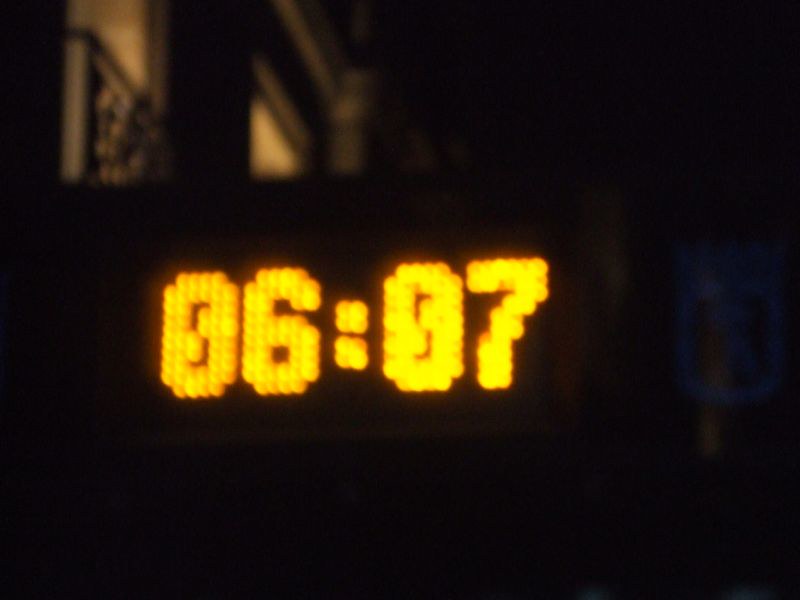This is a nighttime photograph featuring a digital clock mounted on the outside of a building. The clock stands prominently in the center-left of the image, displaying the time as "06:07" in bright yellow lights with an orange hue. The numbers are composed of individual bulbs, reminiscent of an old-fashioned scoreboard clock. Surrounding the clock is an enveloping darkness, with only faint details visible. In the background to the right, there is a barely discernible blueish sign, and above the clock, what appears to be the second story of the building, possibly with windows, faintly illuminated to a bronze-beige color. Shadows are also evident in the upper left corner of the photograph, suggesting the presence of a window or door behind the clock. The image is slightly blurry, adding to the difficulty of making out further details.